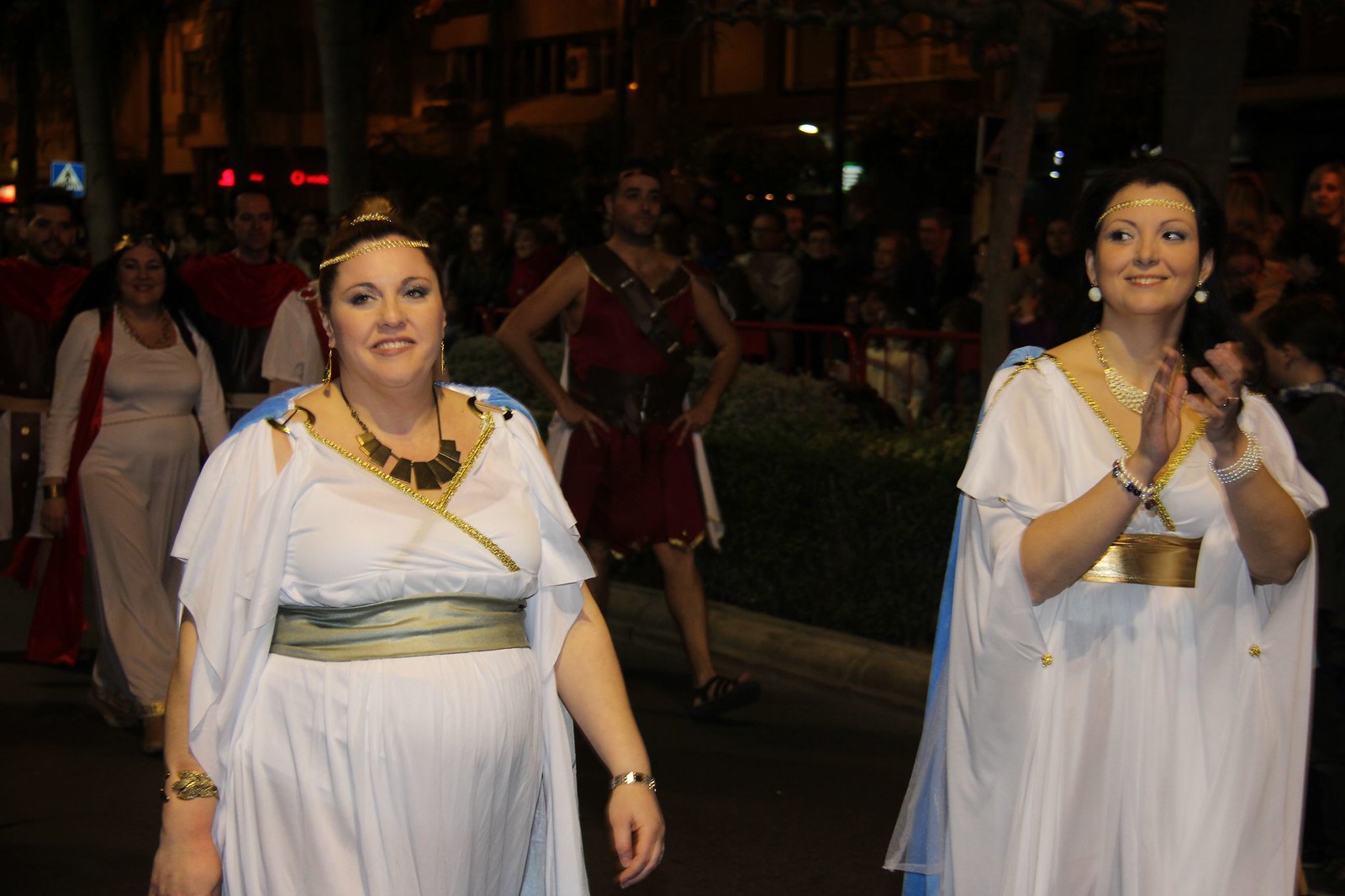This photographic image, taken outdoors at night, captures a parade scene featuring two women in the foreground, dressed in ancient Roman-inspired attire. Both women are wearing long white gowns with gold accents - one has a silver sash while the other has a gold belt. The dresses, reminiscent of togas, feature short sleeves and are adorned with intricate accessories such as long earrings, jade necklaces, and multiple bracelets. The woman on the left is overweight and smiles warmly, while the woman on the right is seen applauding. Behind them, the scene includes other parade participants: a person in a black tunic and skirt with hands on hips, and another woman in white carrying a pocket book. In the background, there's a well-maintained green hedge, a crowd gathered behind a guardrail, and distant buildings, possibly storefronts. The dark setting is illuminated by some white lights and features an indistinct word in red off in the distance.